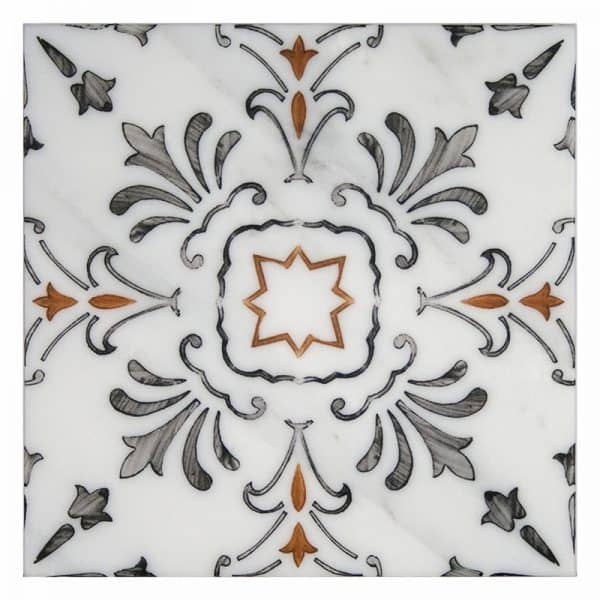This image showcases a meticulously designed decorative piece, possibly a digital creation or artwork, depicting intricate patterns and symmetrical elements. The entire design is encased in a square frame with a white background. At the center lies an eight-pointed star rendered in brown, surrounded by a dark black outline. Extending from this central star, various elements radiate in eight different directions. These elements include four black, fleur-de-lis-like shapes pointing diagonally towards the corners, and four upside-down Christmas tree shapes with orange and black designs oriented perpendicularly. Additional spear-like, angular shapes in black direct towards each corner of the image. The overall composition exhibits a harmonious blend of colors, including shades of gray, bronze, brown, off-white, and black, arranged in a balanced and repetitive pattern that flows outward from the central star, creating a captivating geometric display.